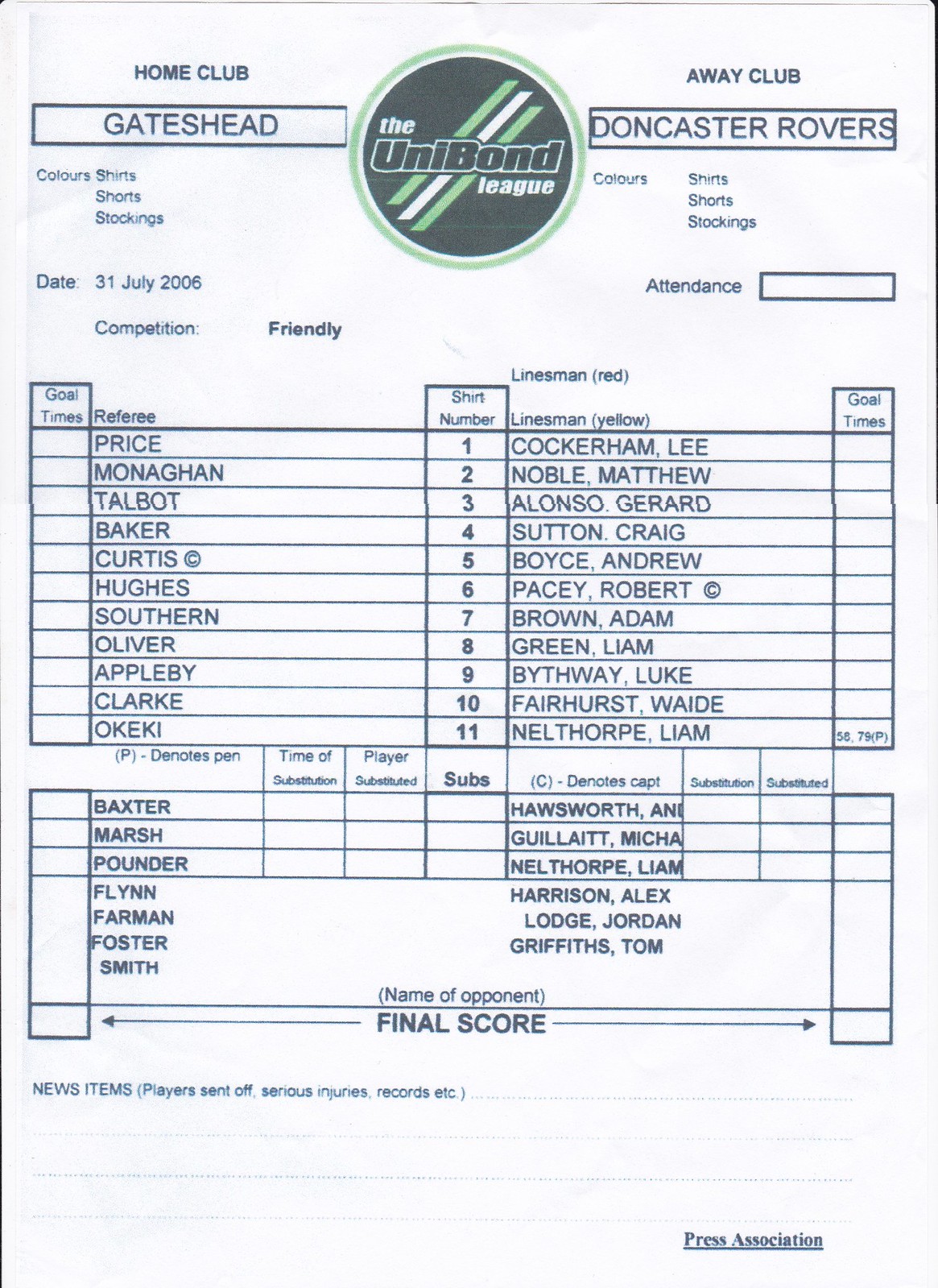This image is a scan of a form, primarily in black and white, designed for documenting a soccer match for the Unibond League. The top features a logo for the Unibond League, distinguished by a dark green circle with a light green outer rim and white text. In the upper left corner, it lists the "Home Club: Gateshead," and in the upper right corner, the "Away Club: Doncaster Rovers." Below these headings, there are sections for team colors, including shirts, shorts, and stockings for both clubs. The date of the match is noted as 31 July 2006, under the heading "Competition: Friendly." There are placeholders for the attendance, final score, and goal times. The form is structured in a grid-like fashion to record detailed information about the players, shirt numbers, and other relevant match details. Noteworthy mentions on the grid include players like Monaghan and Talbot for Gateshead, with a similar list for Doncaster Rovers. Referee information and additional names, possibly substitutes or key roles like captains, such as Baxter, Marsh, and Pounder, are also listed. Certain fields, such as the attendance and final match score, appear to be left blank, suggesting the match has not yet taken place.